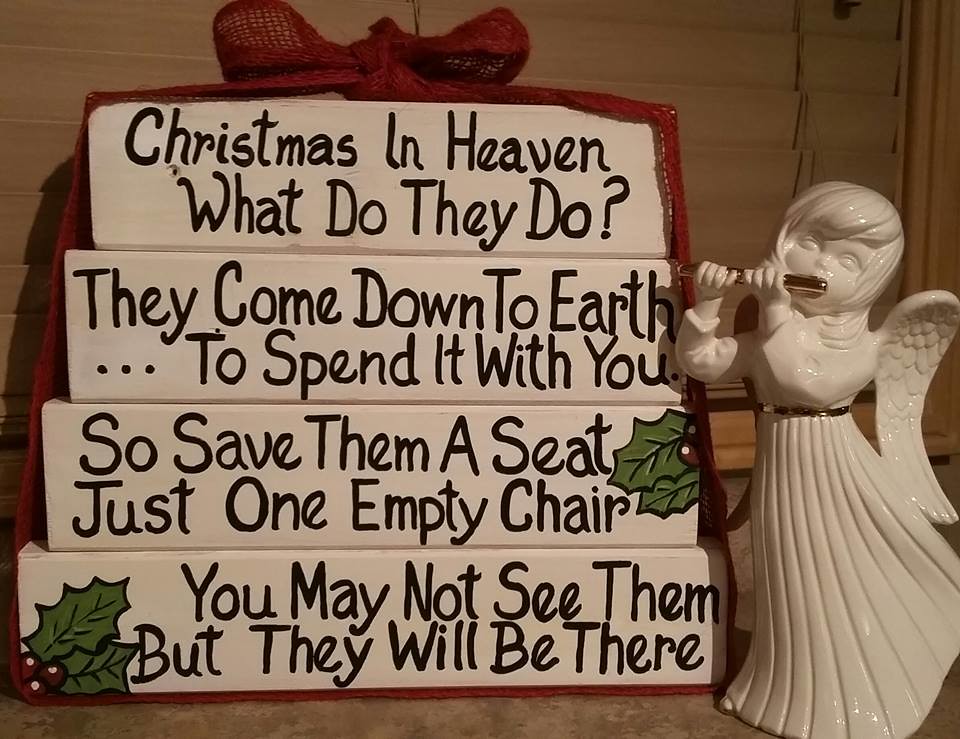In a warm indoor setting, this photographic image captures a touching Christmas decoration scene. At the center stands a delicate porcelain angel statuette adorned in a flowing white robe tied with a black belt, and she plays a golden flute with serene expression while her angelic wings spread gracefully. Beside her are four ceramic blocks arranged vertically, each inscribed with a heartfelt message in black text: "Christmas in heaven, what do they do?", "They come down to earth to spend it with you", "So save them a seat, just one empty chair", and "You may not see them, but they will be there". The blocks are festively adorned with green holly leaves and are topped with a red bow. The background reveals white wooden window blinds, while everything rests on a table, completing this poignant and beautifully arranged festive display.